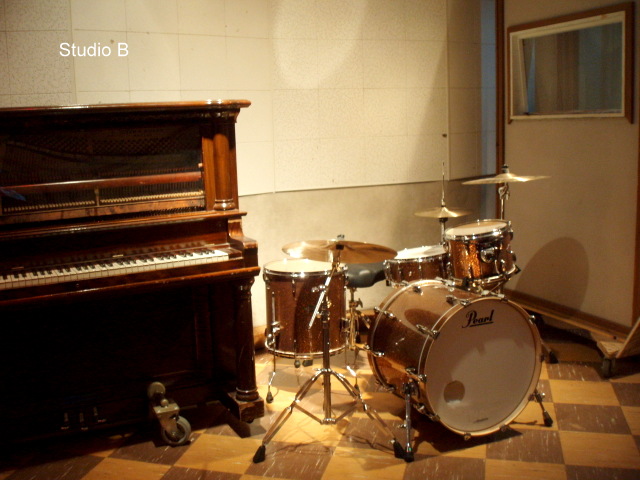The image captures a well-equipped music studio labeled "Studio B" in thin text at the upper left corner. Dominating the left side of the room is an old, wood-toned piano set on wheels. Adjacent to it, centrally positioned, is a Pearl brand drum set featuring a white canvas finish with silver hardware. The drum kit includes a kick drum prominently displaying the Pearl logo, a snare drum, one tom, a floor tom, a hi-hat, a ride cymbal, a crash cymbal, and additional cymbals. The backdrop consists of a white and tan wall with a large window, allowing natural light to enter the space. The floor showcases a distinctive black and white checkerboard pattern, adding to the studio's unique aesthetic.